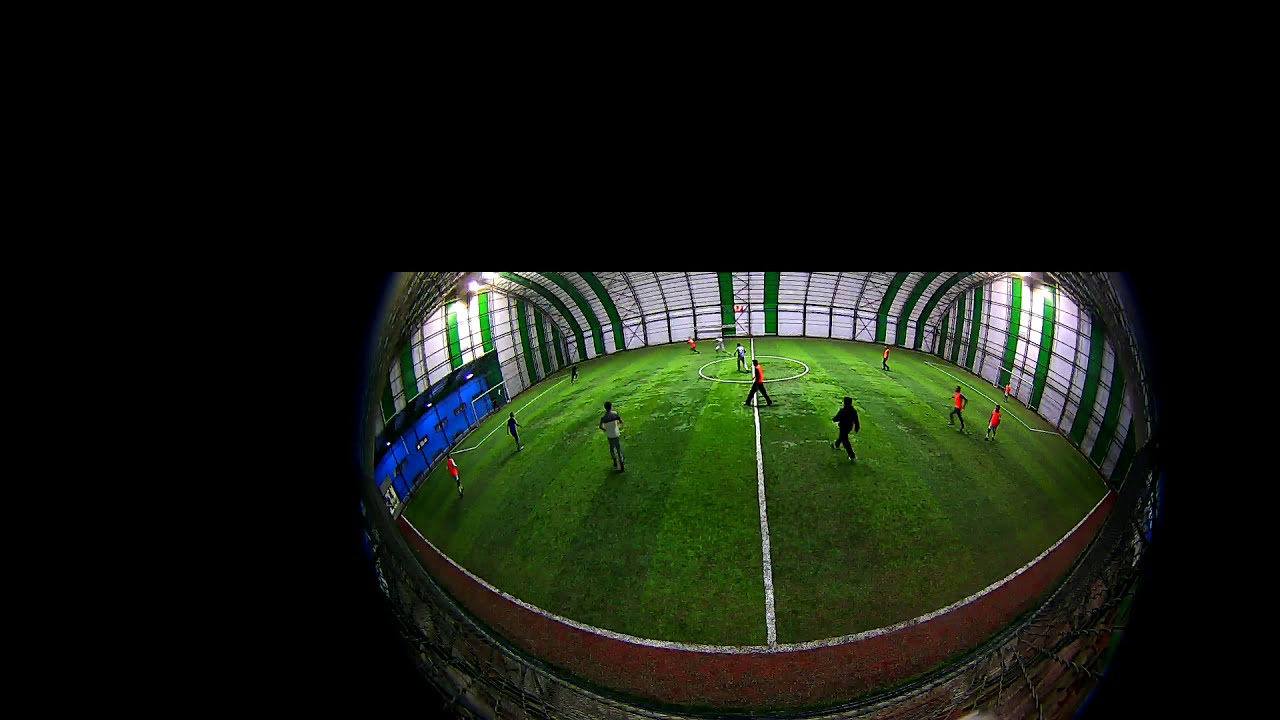This photograph, taken indoors with a fisheye lens, presents a distorted, globe-like view of a soccer field. The green grass is meticulously maintained, displaying alternating dark and light green stripes that enhance the field's aesthetic appeal. The entire area is enclosed by a glass dome, composed of multiple translucent panes that create a semi-dark ambiance. The field is bordered by white and green walls and features blue doors on the left side. At least thirteen players are scattered across the field, wearing a mix of red or orangish shirts paired with white shorts or black leggings, while a few are in black or white shirts and pants. The image also reveals two goals, positioned on the right and left, and a central line running down the middle of the field. The scene lacks spectator seating, with an unobstructed view of metal scaffolding in the corners, adding to the industrial feel of the arena. Despite the graininess of the image, the overall composition effectively captures the vibrant, organized nature of the indoor soccer environment.